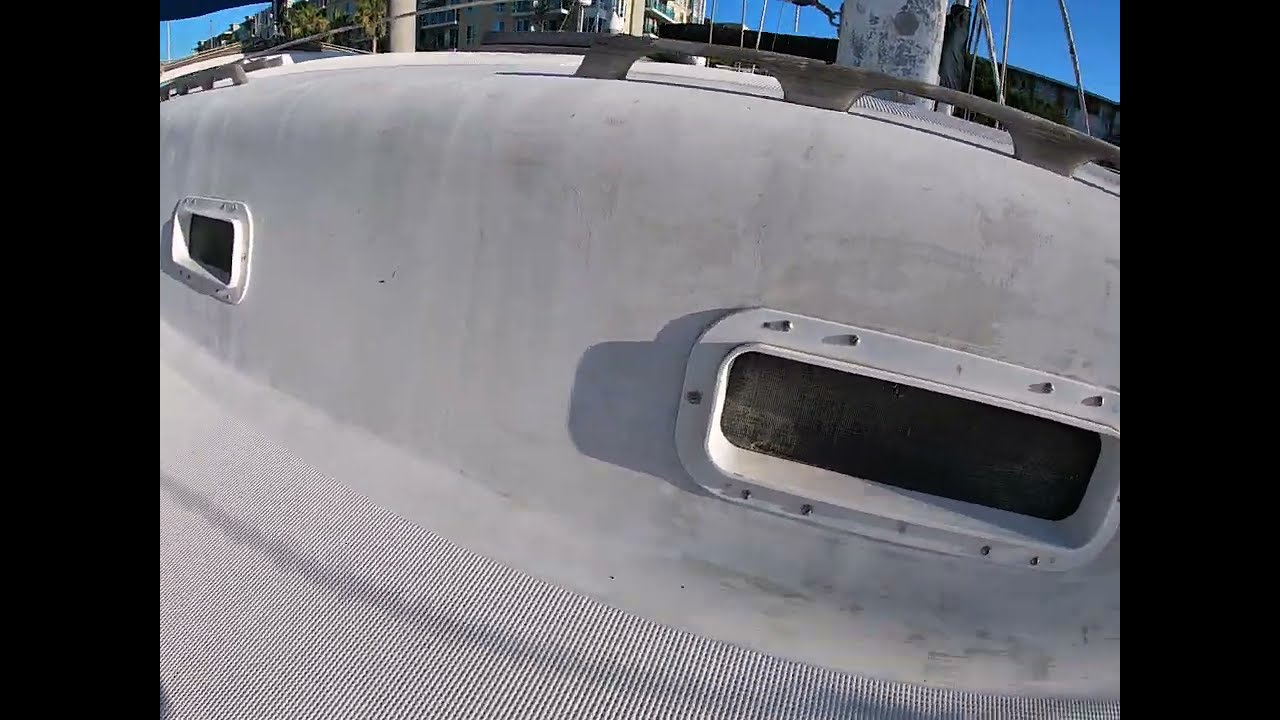The photograph showcases the side structure of what appears to be a bridge or overpass, captured using a fisheye lens that provides a broad, sweeping view. The image is dominated by a concrete surface featuring small, rectangular ports that likely serve as drainage. In the foreground, a railing is prominently visible, giving the impression of a roadway or pavement extending across the scene. The sky is a clear blue, suggesting the photo was taken outdoors during the day. In the background, there's a glimpse of buildings, possibly apartment complexes, contributing to the urban setting. Additional elements such as cables and pulleys hint at the structural supports of the bridge. The overall color palette includes various shades of gray, black, blue, and tan. The entire frame is filled with these contrasting textures and details, with no visible text or signage.